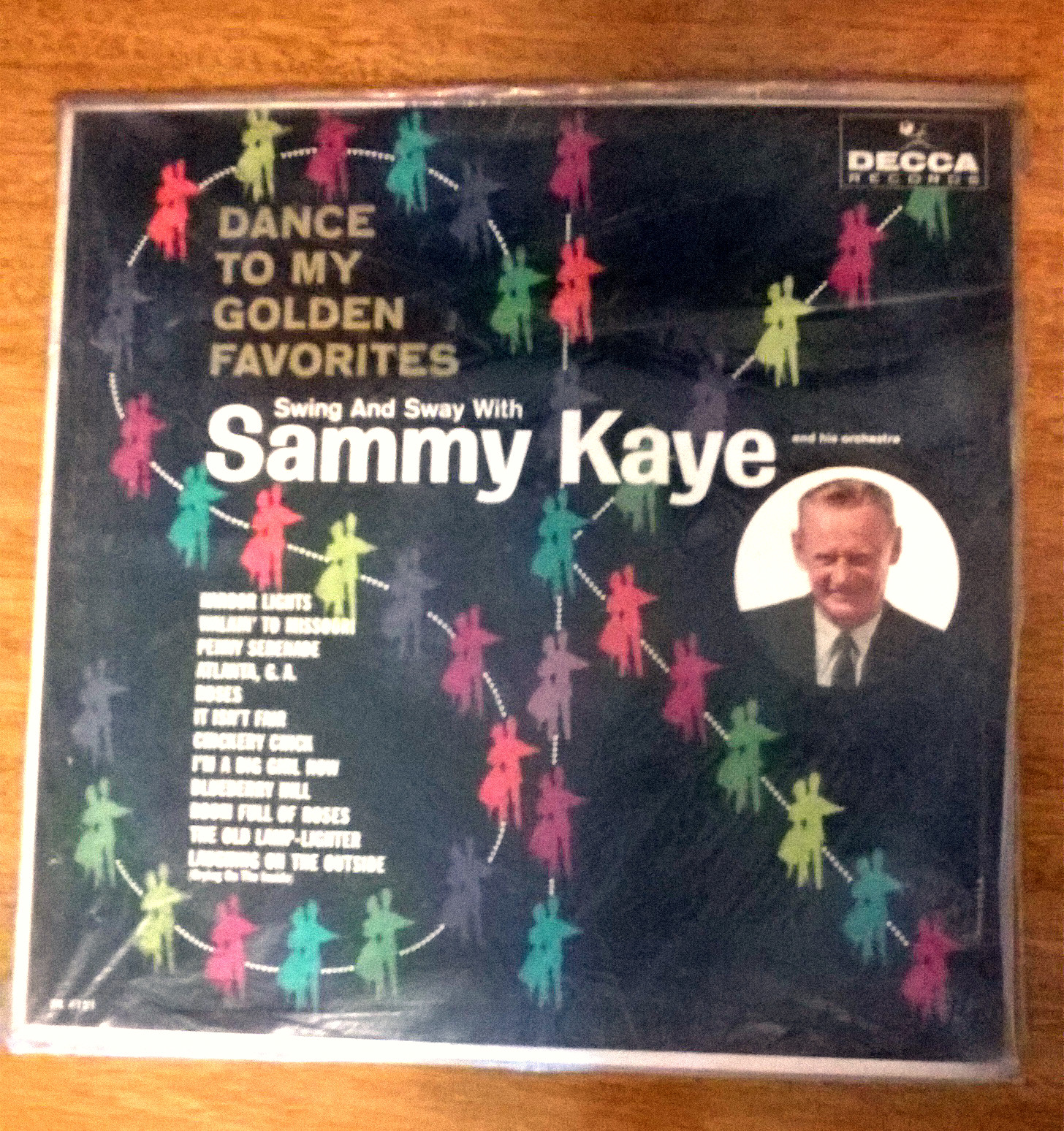This photograph captures a vintage album cover resting on a woodgrain table. The album, titled "Swing and Sway with Sammy Kaye and His Orchestra," prominently features a black background with thin, white outlined letters 'S' and 'K' that nearly fill the cover. These letters are adorned with colorful silhouettes of ballroom dancing couples in hues of blue, yellow, pink, green, purple, red, beige, and light blue, following the shapes of the 'S' and 'K'.

At the center of the album cover, golden text reads "Dance to My Golden Favorites," with the subtitle "Swing and Sway with Sammy Kaye" in white beneath it. A small circular photograph of Sammy Kaye, depicted as an older white man in a suit and tie, is situated off to the right. Above the title, smaller text states "And His Orchestra." 

Though part of the text listing the album's tracks on the lower left is blurry, readable titles include "Indoor Lights, Atlanta, Georgia," "It Ain't Fair," "Crockery Crook," "I'm a Big Girl Now," "Blueberry Hill," and "The Old Lamp Lighter." The album is released by DECA Records, with its label printed on the left side of the cover.